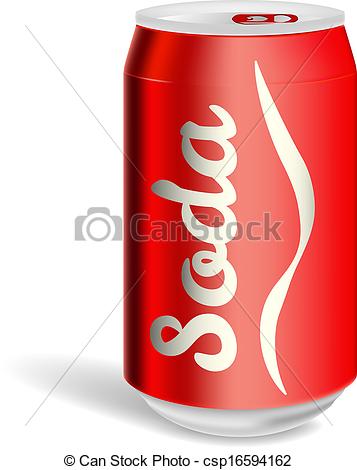This is a stock photo of a red aluminum soda can, reminiscent in style to a Coca-Cola can, but clearly labeled as "soda" in a vertical orientation with a wavy silver line. The can features the typical silver color at the top and bottom, and it includes a red pop tab. Across the entire image, there is a gray X watermark, with a camera icon and the text "Can Stock" superimposed in the center. At the bottom of the image, formal black text reads "Can Stock Photo" with the identification number "CSP 16594162." The can is set against a simple white background.